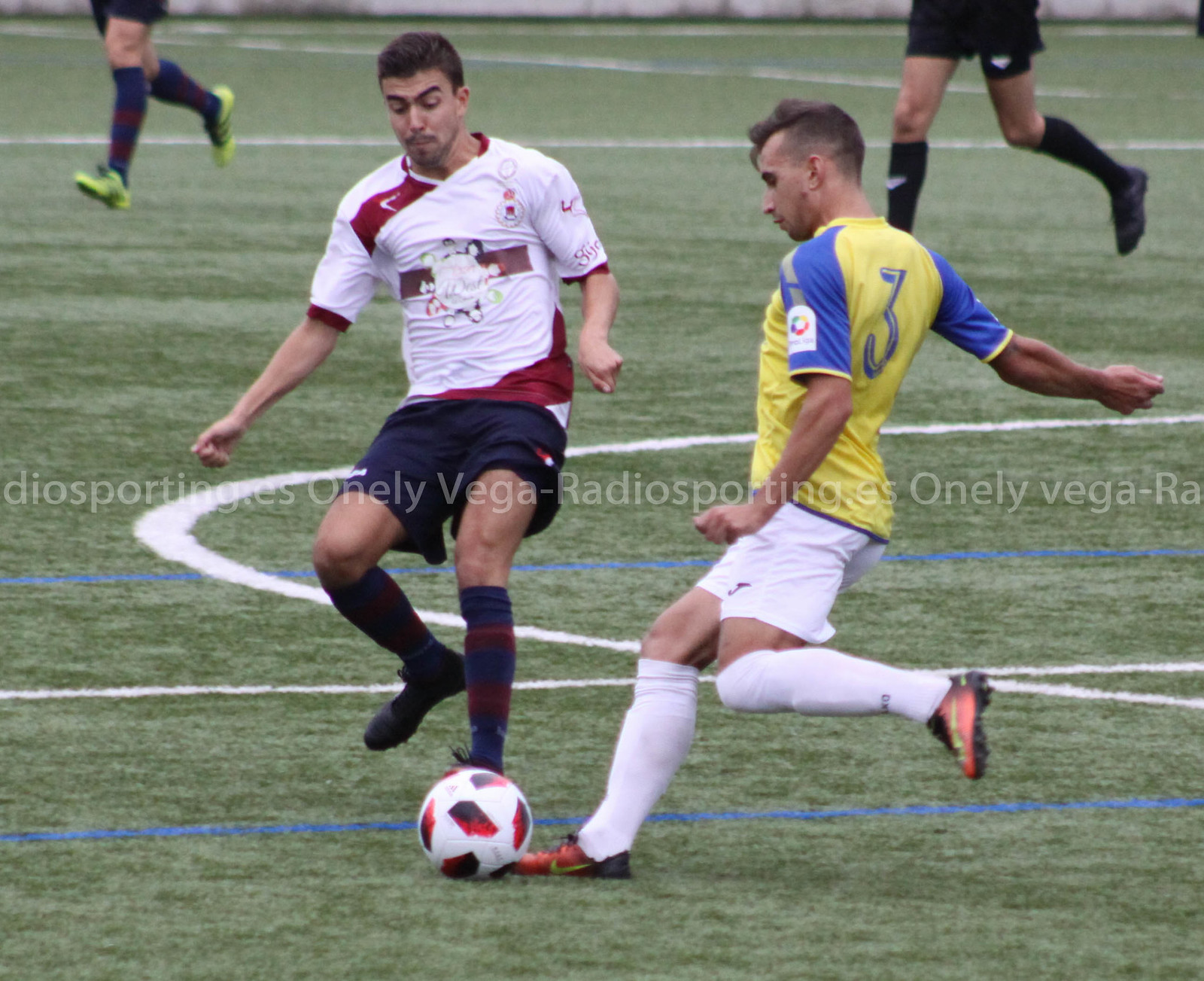The image captures an intense moment of a professional football match in progress, played outdoors during the daytime. Dominating the foreground are two players from opposing teams converging on the ball. One player, with tan skin and dark brown hair, is seen wearing a yellow jersey with blue short sleeves and the number three on his back. He sports white shorts, white socks, and orange soccer shoes with yellow stripes, and is poised to kick the ball. The opposing player, attempting to block the kick, features short brown hair and is clad in a white and purple jersey, navy blue shorts, and blue-and-red socks. The soccer ball, prominently placed between them, is white with black and red patches. In the background, the green field is visible with horizontal blue stripes, white lines, and circles, intertwined with the watermark "Radio Sporting's One Leaf Vega" in transparent white, running across the center. Visible in the upper left and right corners are the lower halves of two additional players racing towards the action.